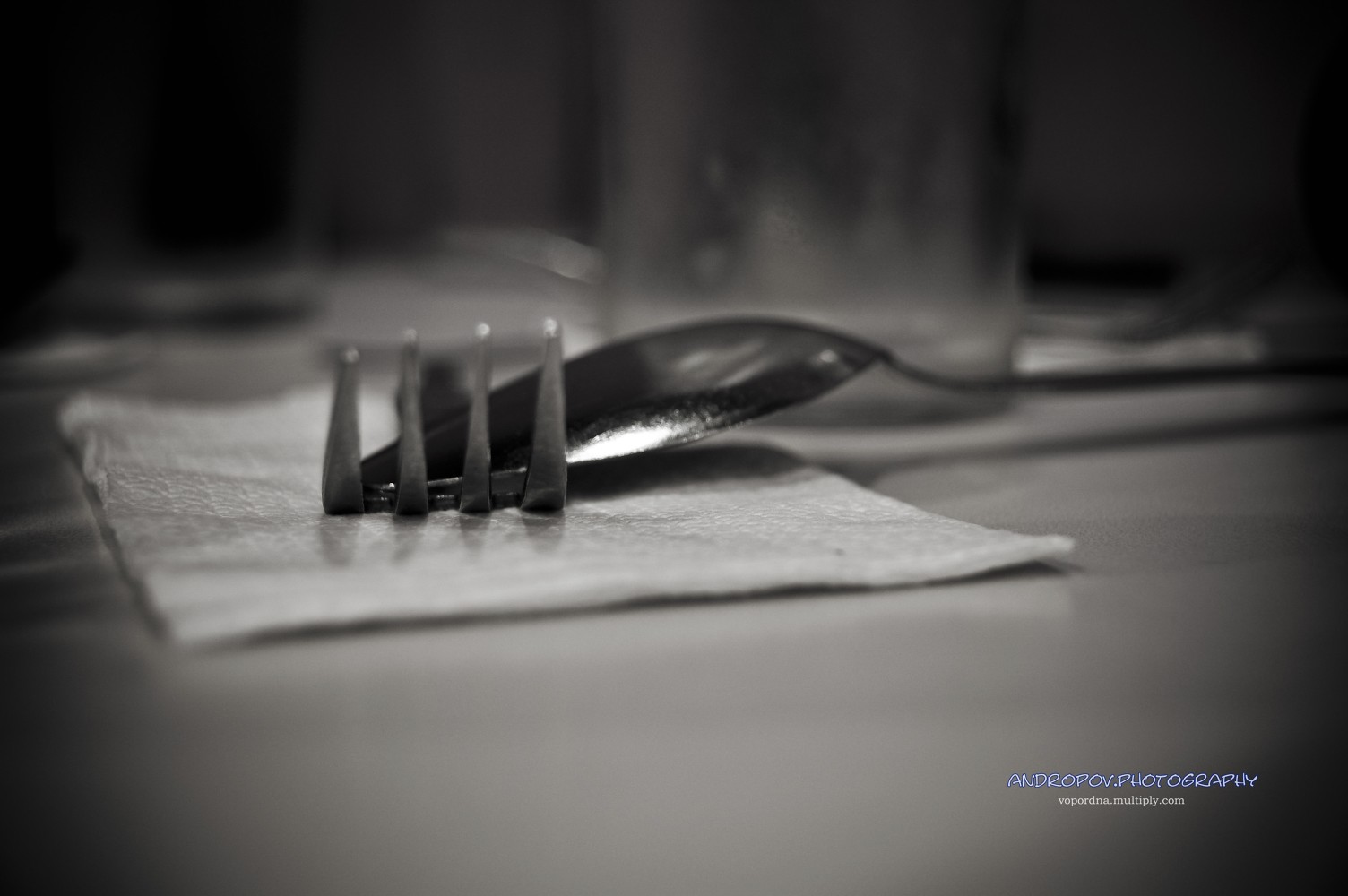This black-and-white artistic photograph captures a detailed tabletop scene. At the center of the composition, a fork lies on its back atop a white paper napkin, with its curved tines facing upwards. Crosswise over the fork is an upside-down spoon, with the handle extending out of the frame. The background, rendered out of focus, hints at a blurry tumbler and additional place settings, suggesting a dining table setting. In the bottom right corner, the image is signed "andropov.photography" in blue font, with "voporna.multiply.com" in white font beneath it, adding a touch of color to the monochrome artwork.